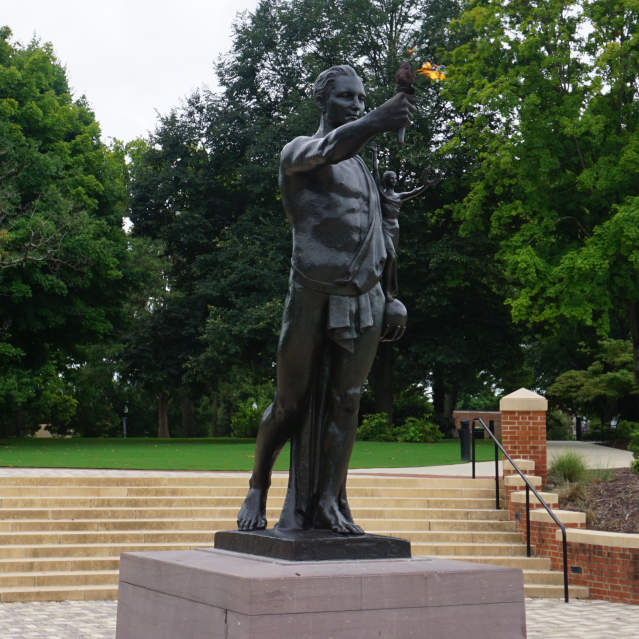The image portrays a prominent statue of a man, intricately detailed and painted a reflective dark black, standing firmly on a gray concrete platform situated in the middle of a well-manicured park. The figure is depicted wearing a minimal toga-like sheath around his waist, with a cape draped over one shoulder, revealing the muscular contours of his body, including his bare feet. In his right hand, he holds aloft a torch with a flame, which seems to evoke an Olympic theme. Below the statue, the ground is paved with white bricks, extending to an area that leads to a small pavered courtyard. Behind the statue, a series of approximately ten cement steps ascends to a higher grassy area, which is meticulously mowed and bordered by numerous beautiful trees. A pathway beyond the steps meanders toward the tree-covered background, adding further depth to the serene daytime scene under a white sky. Moreover, a brick retaining wall is present, housing a flower garden that adds to the idyllic park atmosphere.